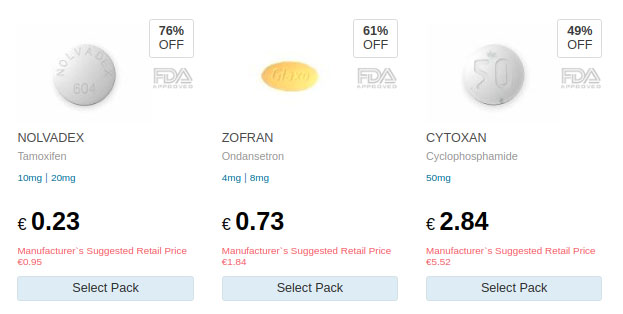This screenshot showcases three different pharmaceutical products available on an e-commerce website, each prominently displayed with details about discounts, dosages, and prices. 

**Product 1: Novadex**  
- **Description:** Novadex is a white, circular pill stamped with "Novadex" and "604." It is FDA-approved and contains Tamoxifen.  
- **Dosage Options:** Available in 10 mg and 20 mg variants.  
- **Pricing:** Currently offered at €0.23 per pill, marked down significantly from the manufacturer's suggested retail price of €0.95, reflecting a 76% discount.  
- **Packaging:** Select Pack available.

**Product 2: Zofran**  
- **Description:** Zofran comes in a yellow, oval shape and is prominently advertised with a 61% discount.  
- **Dosage Options:** Available in 4 mg and 6 mg variants.  
- **Pricing Details:** Not specified in the text.

**Product 3: Cytosan**  
- **Description:** Cytosan is another white, circular pill, marked with "50."  
- **Dosage Option:** Available exclusively in a 50 mg variant.  
- **Other Information:** Pricing and discount details are not specified within the text.

Each product includes various attributes appealing to consumers, such as significant discounts and clear dosage information.